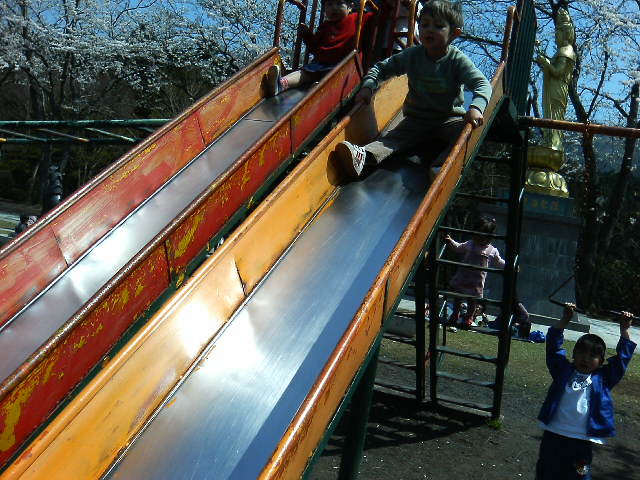In the foreground of the photo, occupying the left two-thirds of the image, are two parallel metal slides with silver centers—one with red rails on the left and one with yellow rails on the right. The paint on the slides is worn; on the red slide, yellow paint is visible through the chipped areas, and on the yellow slide, red paint shows through the worn spots. Each slide has an accompanying ladder leading to the top. At the top of the slides are two children: the child on the red slide wears shorts and a red shirt, preparing to descend, while the child on the yellow slide, already beginning to slide down, wears a blue shirt, long pants, and white shoes with red stripes. 

To the right of the slides, another child hangs from triangle-shaped bars extending horizontally from a jungle gym structure that also includes a green monkey bar ladder. In the background, a large pedestal with a golden statue facing left stands prominently. The trees around are budding, adorned with white blossoms, indicating early spring. Several people are seated on the grass, blurred out by the slide ladders, adding to the lively playground atmosphere. The blue sky completes this joyful scene, filled with children playing and vibrant nature.